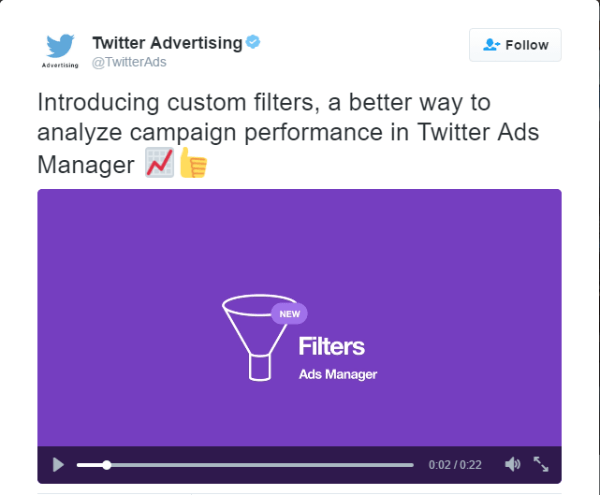Here is a more detailed and cleaned-up caption for the described image:

---

This advertisement, designed for a cell phone screen, prominently features the classic blue bird logo of the former Twitter platform in the upper left corner. Beneath the logo, "advertising" is written in small black font. "Twitter Advertising" appears in larger black font next to the bird, with the handle "@TwitterAds" just below it, accompanied by a follow button and a blue verification checkmark.

The central message reads: "Introducing custom filters, a better way to analyze campaign performance in Twitter Ads." Adjacent to this, there's an icon indicating a manager role, depicted as a white square with a red arrow or trending line pointing upwards. Below that is a yellow thumbs-up emoji.

At the bottom portion, there is an embedded video provided by Twitter, detailing the functionality of the new filters and the ad management system. Users can click on the video to learn more about these features.

---